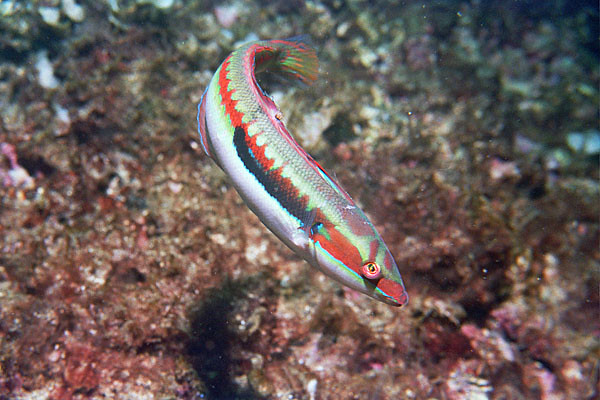This underwater photograph features a long, slender fish swimming gracefully above a coral reef. The coral backdrop showcases a blend of brown, reddish, and some purplish hues. The fish itself is striking, adorned with a kaleidoscope of colors: a white belly, a prominent red stripe running from its nose past its eye and down its side, overlaid by a smaller black band near its gills. Further along its body runs a green band, with gray adorning its dorsal side. The fish's eyes are notably red and black. Positioned centrally in the frame, the fish's tail is delicately curved to the right, emphasizing its elegant motion through the ocean waters.